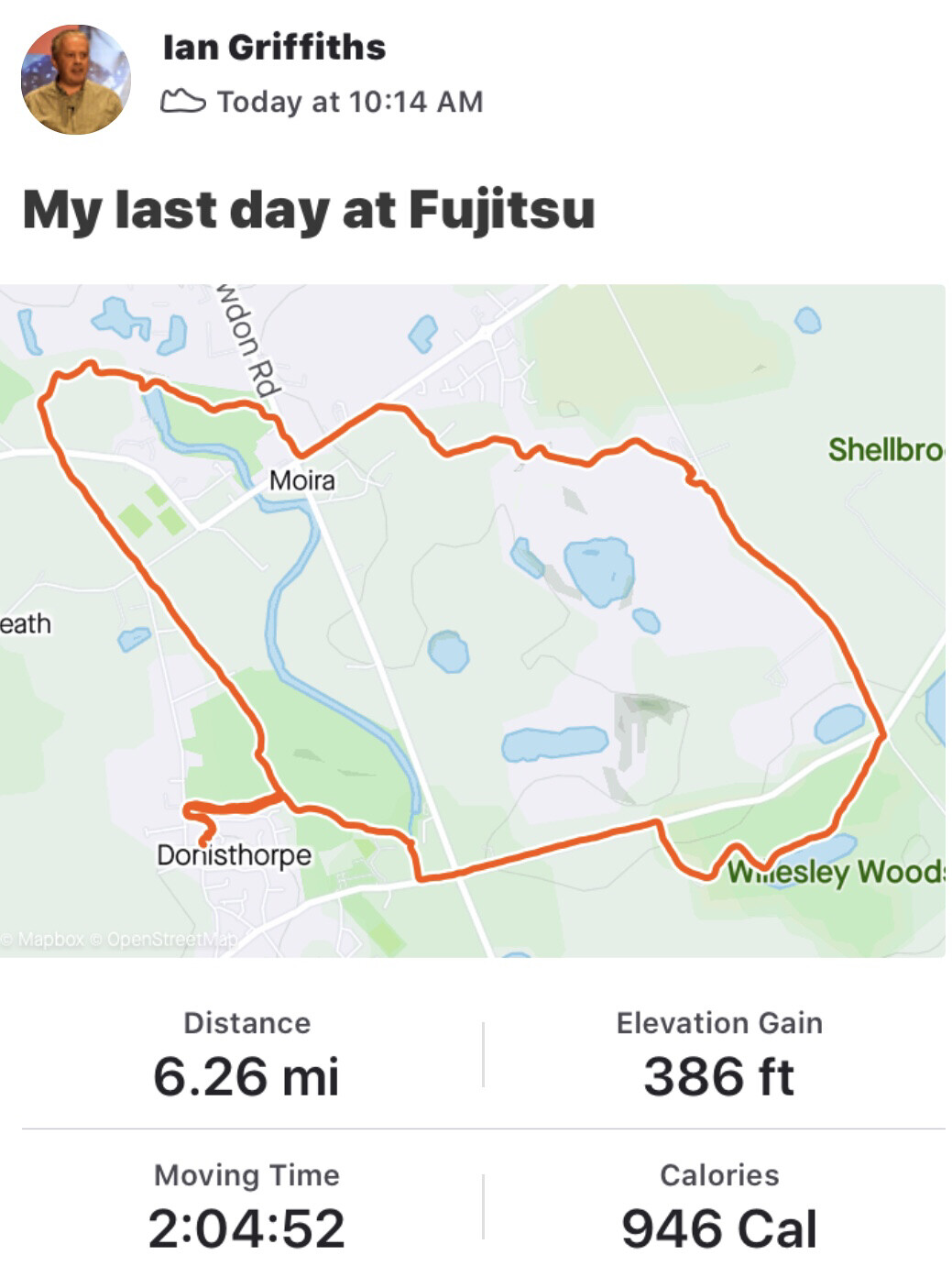Ian Griffiths posted on social media today at 10:14 a.m., marking his last day at Fujitsu. His profile picture, a small circular icon, shows a white man in his late 40s or early 50s, wearing a mustard-colored shirt, with a blue and red background. Next to his name, a shoe icon denotes a fitness activity. The post features a map with a route highlighted in red, connecting various locations including Moira at the top and Donisthorpe at the bottom. The route details indicate a distance of 6.26 miles, an elevation gain of 386 feet, a moving time of 2 hours, 4 minutes, and 52 seconds, and a total calorie burn of 946 calories.